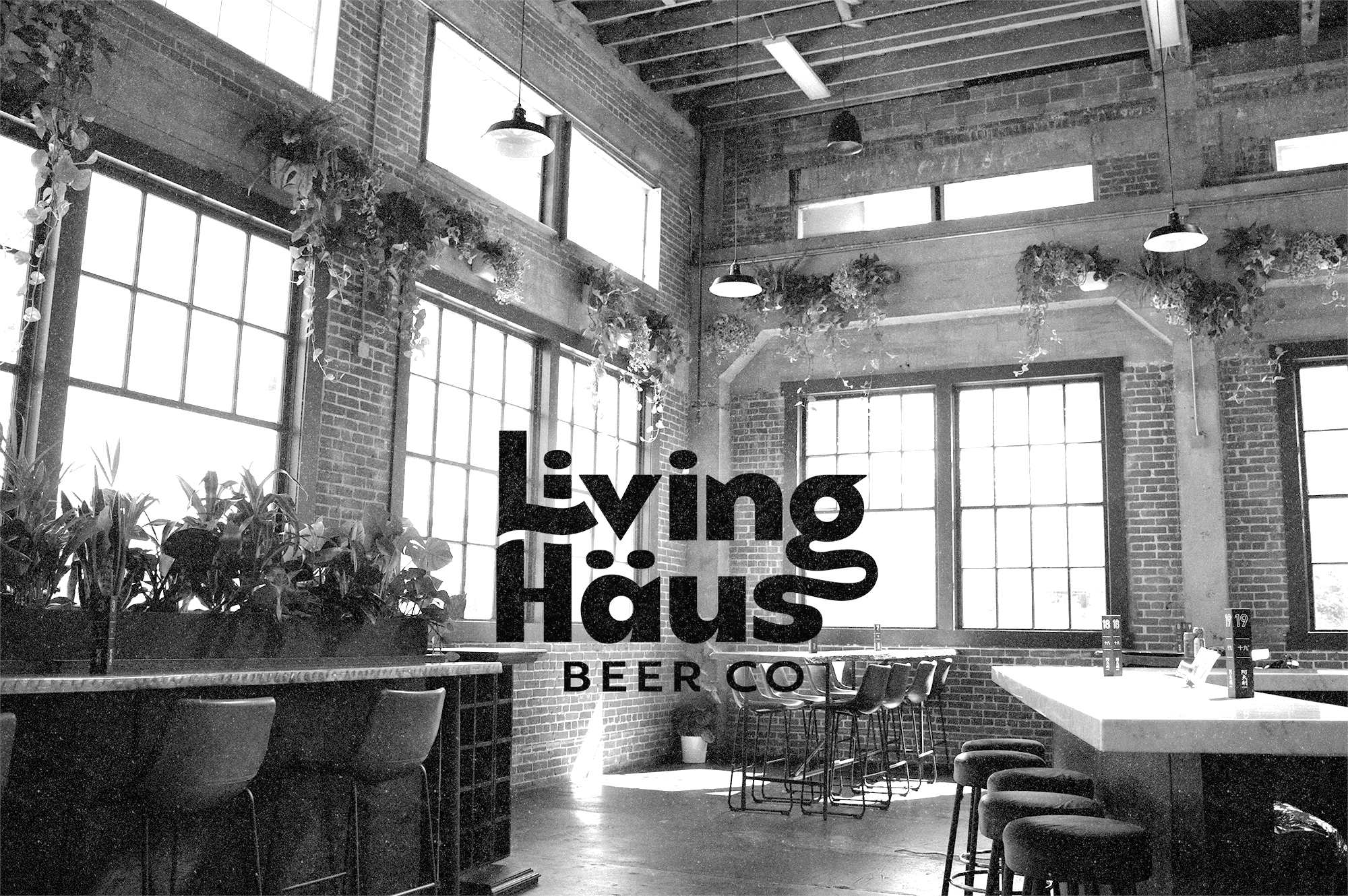This black and white photo captures the interior of Living Haas Beer Company, a brewery housed in a converted old mill building. The expansive space features high ceilings with exposed wooden beams and large factory-style windows, which flood the room with natural light. The brewery's industrial aesthetic is softened by abundant greenery, including plants hanging down from high above a series of large windows and decorating various corners and railings. The interior showcases a blend of concrete and brick walls. There are high-raised tables with white marble tops, accompanied by a mix of stools and benches for seating. An L-shaped bar with a marble countertop and bar stools is prominently positioned on the right side of the image. Factory-style industrial lights hang down throughout the space, enhancing the modern yet rustic atmosphere. In the center of the image, the words "Living Haas Beer Company" are prominently displayed, branding the inviting and bustling environment.